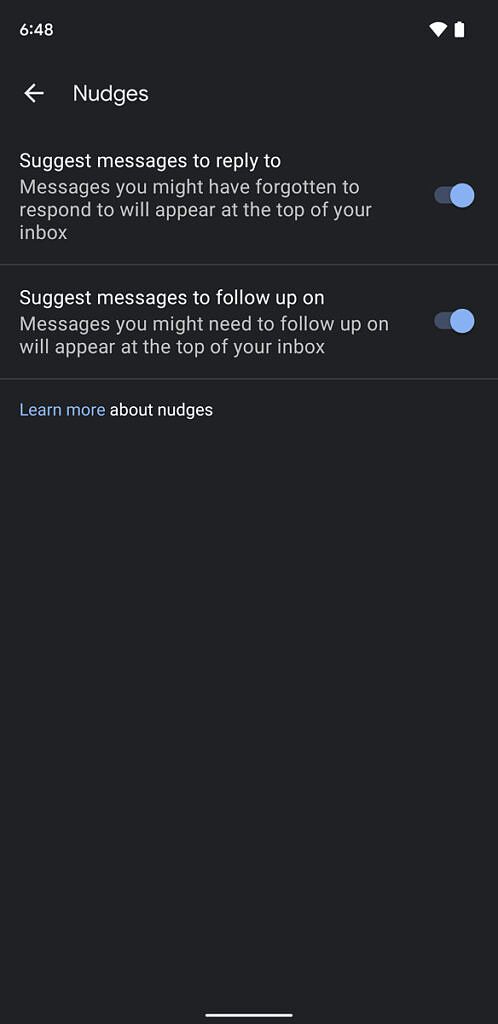The image appears to be a screenshot from a mobile device displaying a settings menu with a black background and white font. At the top left corner, the time reads "6:48," accompanied by icons for Wi-Fi and battery status to the right, all in white.

Beneath this header, the interface shows several settings options related to managing message notifications:

1. The first section features a setting labeled "Nudges" with a leftward-pointing white arrow.
2. The subtitle reads "Suggest messages to reply to," indicating a feature that highlights messages one may have forgotten to respond to, positioning them at the top of the inbox. A blue circle icon to the right suggests this feature is currently enabled.

Following a dividing gray line is another setting:
1. It reads "Suggest messages to follow up on," which highlights messages that might need follow-up actions and similarly places them at the top of the inbox. This too has a blue circle icon to the right, signifying it's activated.

Another gray line below this leads to a link:
1. In blue text, it says "Learn more," followed by "about nudges" in white, guiding users to additional information. A white dividing line is also visible underneath this section.

Notably, each blue circle is nested within a gray outline circle, indicating their interactive element within the settings menu. The layout is spaced generously, providing clear visual separation between each section and icon.